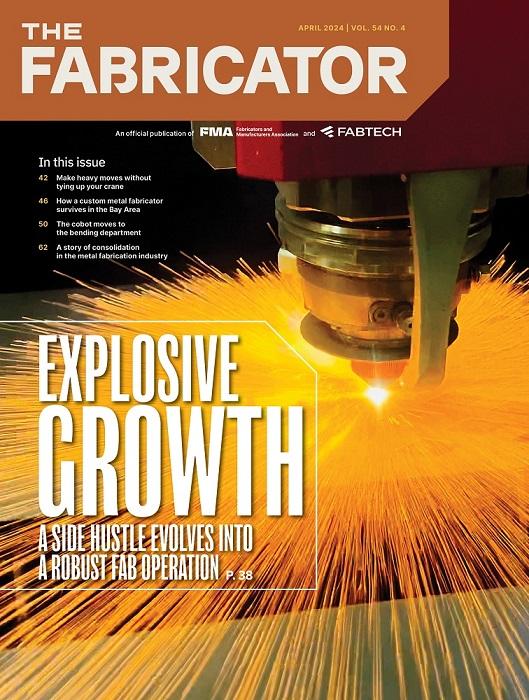The cover of the April 2024 issue of "The Fabricator," volume 54, number 4, an official publication of FMA Fabtech, prominently features a scene of dynamic metalworking. Centered slightly to the right, a robust piece of fabrication machinery emits vivid sparks that spread across the middle of the image, highlighting the intense activity. The rich color palette of orange, yellow, tan, red, brown, white, and black enhances the visual impact, capturing the industrial vibe. The cover text teases exciting articles such as "Make Heavy Moves Without Tying Up Your Crane," "How a Custom Metal Fabricator Survives in the Bay Area," "The Cobot Moves to the Bending Department: A Story of Consolidation in the Metal Fabrication Industry," and "Explosive Growth: A Side Hustle Evolves into a Robust Fab Operation." These headlines complement the dramatic visual, offering a glimpse into the latest trends and stories in metal fabrication.